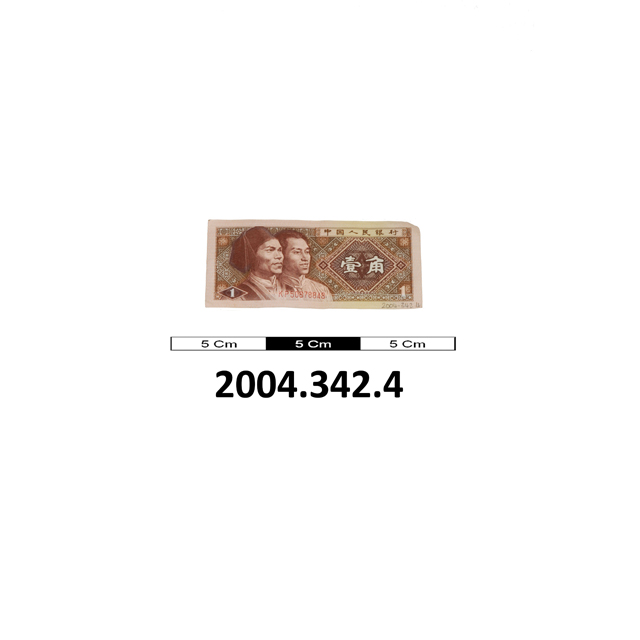The image depicts a close-up of foreign paper currency, likely from an Asian country, characterized by its tan color and rectangular shape. Dominating the left side of the bill are the images of two men with dark hair, both looking towards the right. The background of the image is white. In the corners of the bill, specifically the bottom left and bottom right, the number "1" is prominently displayed inside diamond shapes. The top right corner features a small white box filled with Asian script, which runs horizontally. Beneath the currency, there is a detailed measurement overlay, consisting of a long, thin horizontal rectangle. This rectangle is white, outlined in black, and labeled with the text "5CM" at three intervals: left, center, and right. Additionally, under the "5CM" markings, the label "2004.342.4" is present, though its significance is unclear. The clean and precise details in the image suggest it is a methodical presentation, possibly for cataloging or educational purposes.